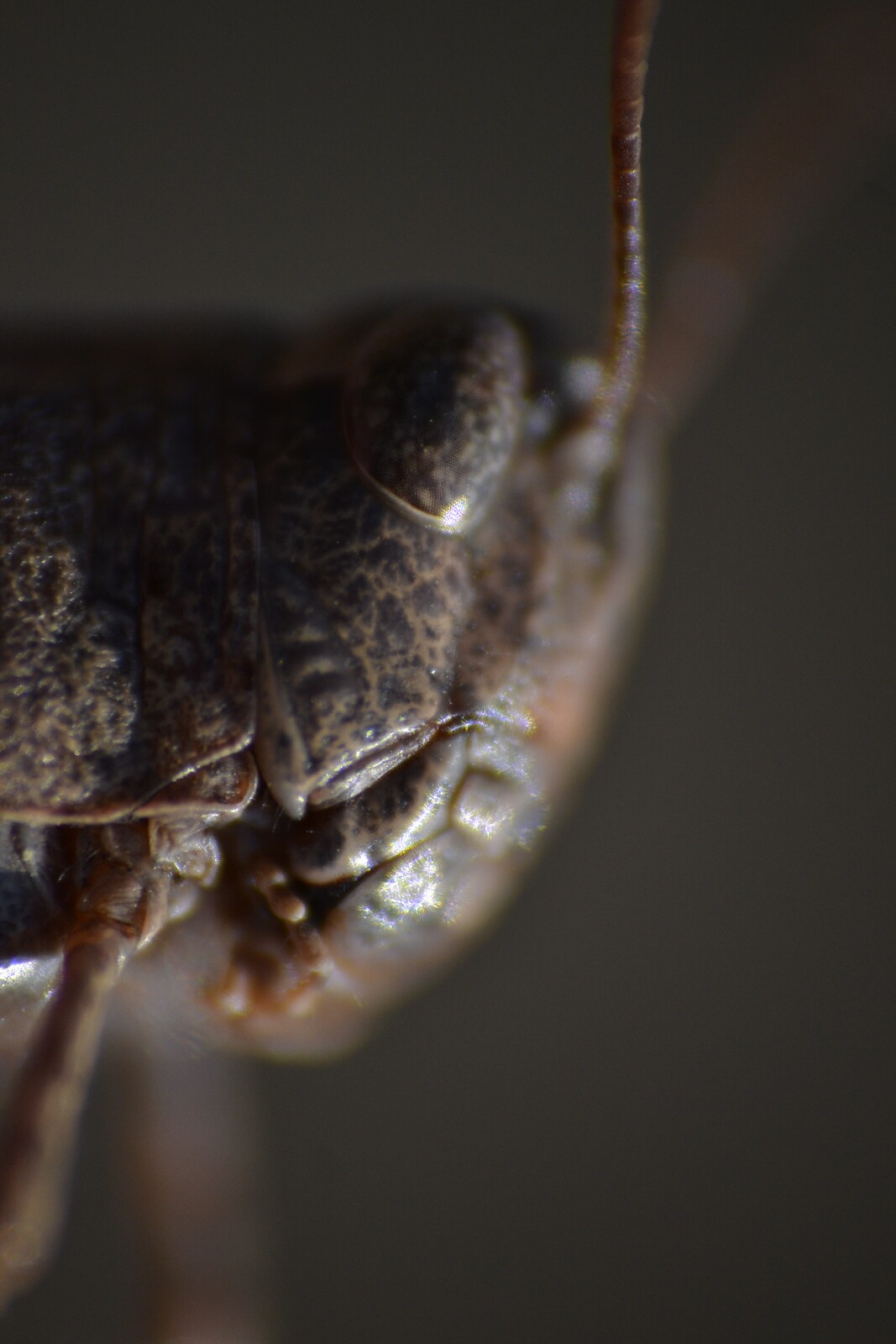This close-up photograph features a magnified view of what appears to be an insect, potentially a grasshopper or a similar bug. The creature's carapace is mottled with brown and black spots, giving it a slightly skeletal or crustacean-like appearance. The picture focuses prominently on the head of the insect, which is framed by antennas or legs protruding from both the top and bottom of the frame. The edges of the image are somewhat blurry, adding to the mysterious quality of the figure. The background is a dark gray, with a slight illumination highlighting the subject, creating a stark contrast between the insect and its surroundings.